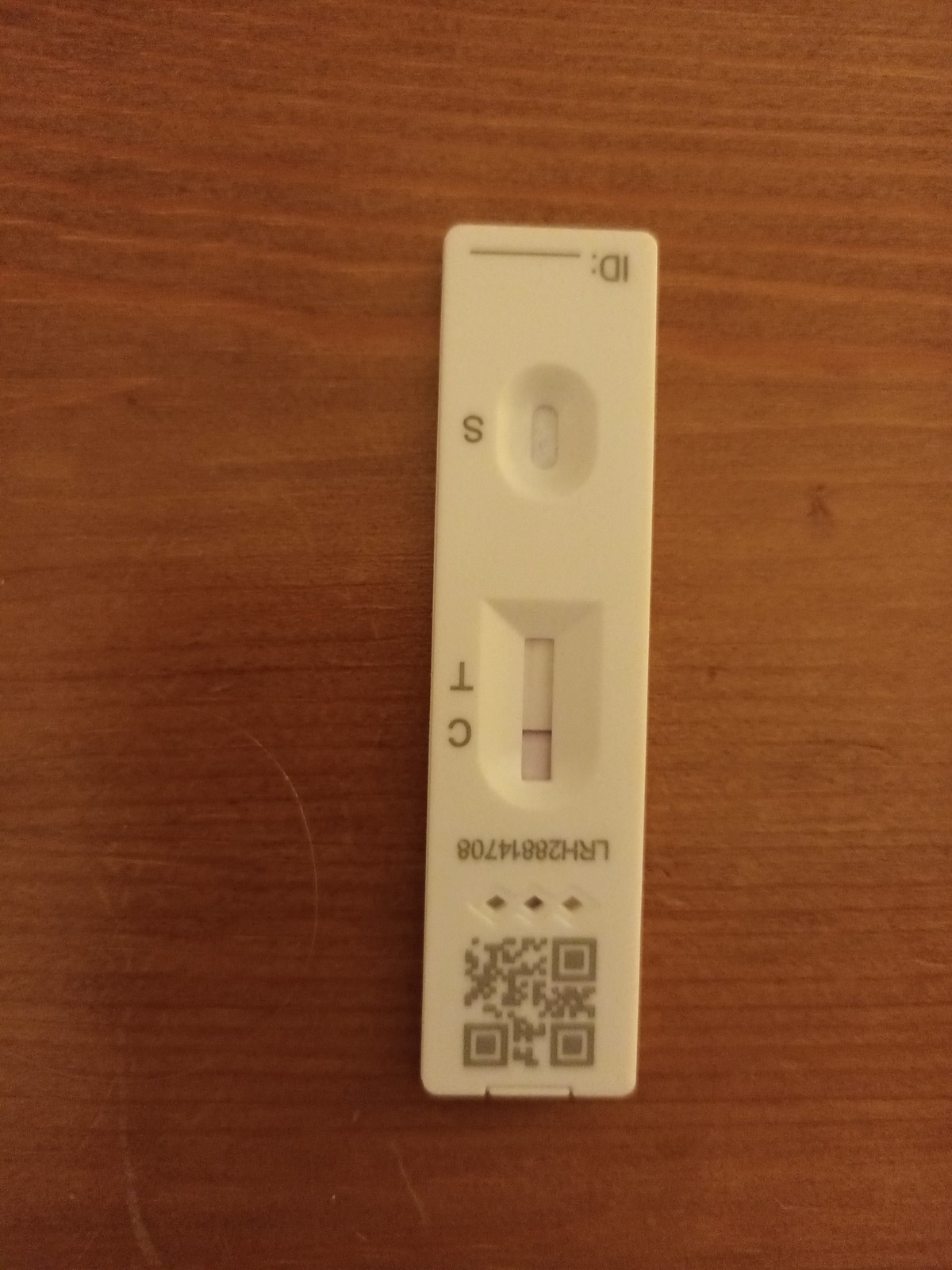This photograph captures an upside-down COVID-19 rapid antigen test lying on a medium-toned brown wooden tabletop. The white test kit is specifically oriented with its QR code positioned at the bottom due to its inverted placement. The test features a rectangular window labeled with 'C' and 'T,' where a single line appears next to the 'C,' indicating a negative result. Below this, an oval window labeled 'S' is present, currently showing no lines. Additionally, there is an area designated for an ID number, though it remains blank in this image. A serial number is visible between the QR code and the rectangular result window, adding an additional layer of identification for the test.